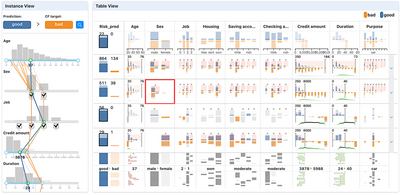This is a visually structured image showcasing a screenshot of a collection of graphs and data tables. The image appears to be cropped, leaving only the titles and the collection of graphs visible. On the right side, there is a distinctive vertical column with a light blue header that reads "Increase View" in bold black font at the top left. Just below this header, there are two buttons, one blue and one orange, separated by an arrow pointing to the right. Above each button, there are small black words that are difficult to read due to the image being minimized and out of focus.

On the left side of the screenshot, there is a vertical sequence of graphs displayed. The first graph at the top is a bar graph labeled "Age" in the top left corner. Below it, there is another bar graph labeled "Sex." The third graph represents "Job," followed by "Credit Amount" as the fourth graph, and "Duration" as the fifth graph.

Dominating the right side of the screenshot is a large box titled "Table View" at the top. Within this box, categories such as Age, Sex, Job, Housing, Checking, Credit Amount, Duration, and Progress are listed across the top. Highlighting a specific section, a graph under the "Sex" category in the third row is emphasized with a red box around it, indicating it has been edited or selected for attention.